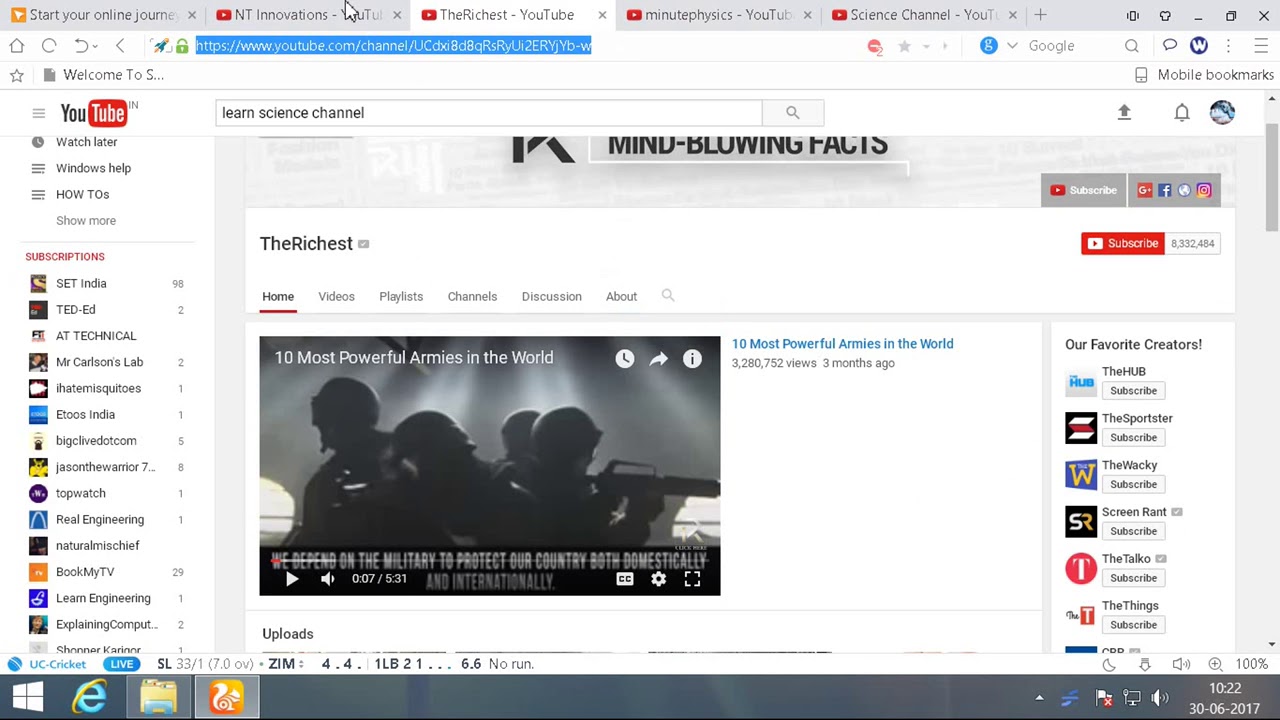A screenshot of a web browser showcases a web page with several open tabs at the top. One prominent tab reads "Start Your Online Journey" inside an orange square box. Another tab labeled "NT Innovations" contains a YouTube video, over which the cursor is hovering. The currently active tab features a YouTube video from "The Richest," playing a video titled "10 Most Powerful Armies in the World." The video is 7 seconds into its total runtime of 5 minutes and 31 seconds, depicting a group of four men wearing helmets and holding AR rifles in a dark environment. Social media buttons for Facebook and Instagram are visible, along with a prominent red "Subscribe" button. Below the video, there are recommendations for various other creators including "The Hub," "The Sportster," "The Wacky," "Screen Rant," "The Taco," and "The Things." At the bottom of the screen, icons for Windows, Internet Explorer, a files button, and an orange squirrel-like logo are displayed. The screenshot is timestamped 10:22 AM on June 30, 2017.